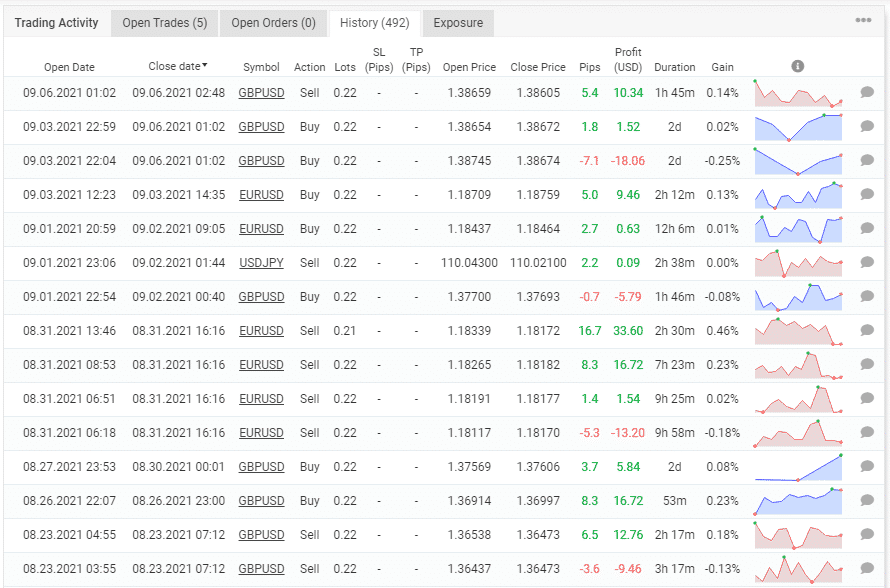A detailed screenshot of a desktop trading application, resembling a spreadsheet, is showcased. The interface features a predominantly white background filled with at least 10 to 15 rows of black text. Notably, two columns distinguishably highlight profits in green and losses in red. Each row is supplemented with small graphs at the far right, depicting the performance fluctuations of individual trades. 

At the top of the interface, a series of tabs provides navigational options, including "Trading Activity," "Open Trades" (with a count of five), "Open Orders" (noting zero), "History" (indicating 492 entries), and "Exposure." The highlighted tab is "History," although "Trading Activity" also appears differentiated, suggesting possible dual focus. 

The "History" tab reveals an extensive log of past trades, with columns detailing the open date, close date, type of action (buy or sell), opening price, closing price, duration, and percentage gain. Each row comprehensively records a historical trade executed by the user, with pertinent data such as pips and profit in US dollars included. The plain aesthetic of the application is accentuated by the vivid green and red indicators of financial outcomes and the arresting mini-graphs summarizing individual trade trajectories.